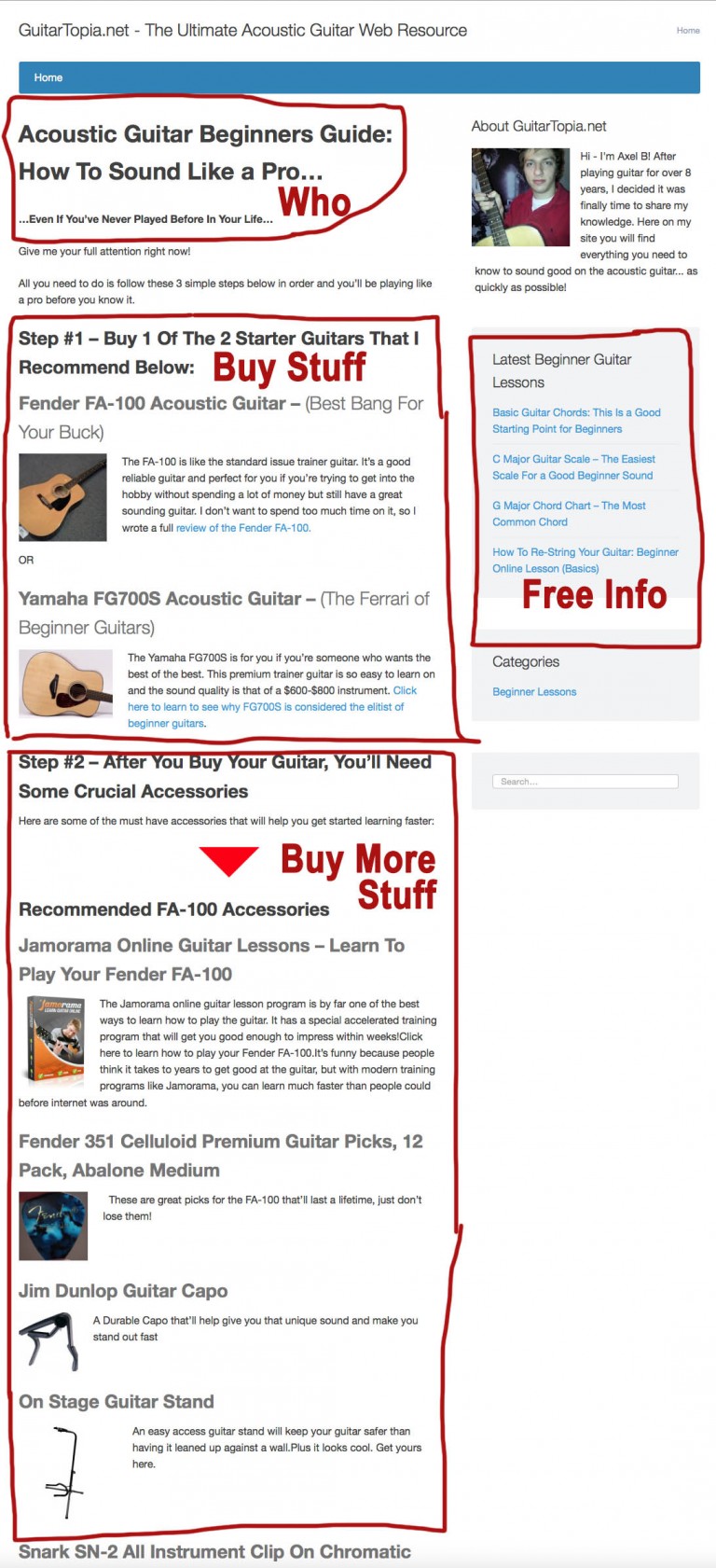**Detailed Caption:**

The image shows a somewhat blurred printout of a webpage from Guitartopia.net, widely recognized as the ultimate acoustic guitar resource. Dominating the top is a distinctive blue bar beneath the title, marking the site's header. Highlighted within the main content are various articles, though the detailed text is unreadable. The article titles remain legible, starting on the top left with "Acoustic Guitar Beginner's Guide - How to Sound Like a Pro," which has been circled in red ink with the word "who" typed beside it. 

Following this on the right, another section begins with "Step 1: Buy one of the two starter guitars that I recommend below," where "buy stuff" is boldly typed in red and encircled. Progressing further right, "Step 2: After you buy your guitar, you'll need some crucial accessories," similarly has "buy more stuff" circled and marked in bold red letters. Although more information is present in these sections, the text isn't clearly visible.

To the far right of the page, there's a photo of a man donning a red sweater. Above his image, the heading "About Guitartopia.net" appears, seemingly containing a personal introduction. Directly below his photo, a box labeled "Latest Beginner Guitar Lessons" is present, encircled in red with the phrase "free info" prominently typed in bold red script.